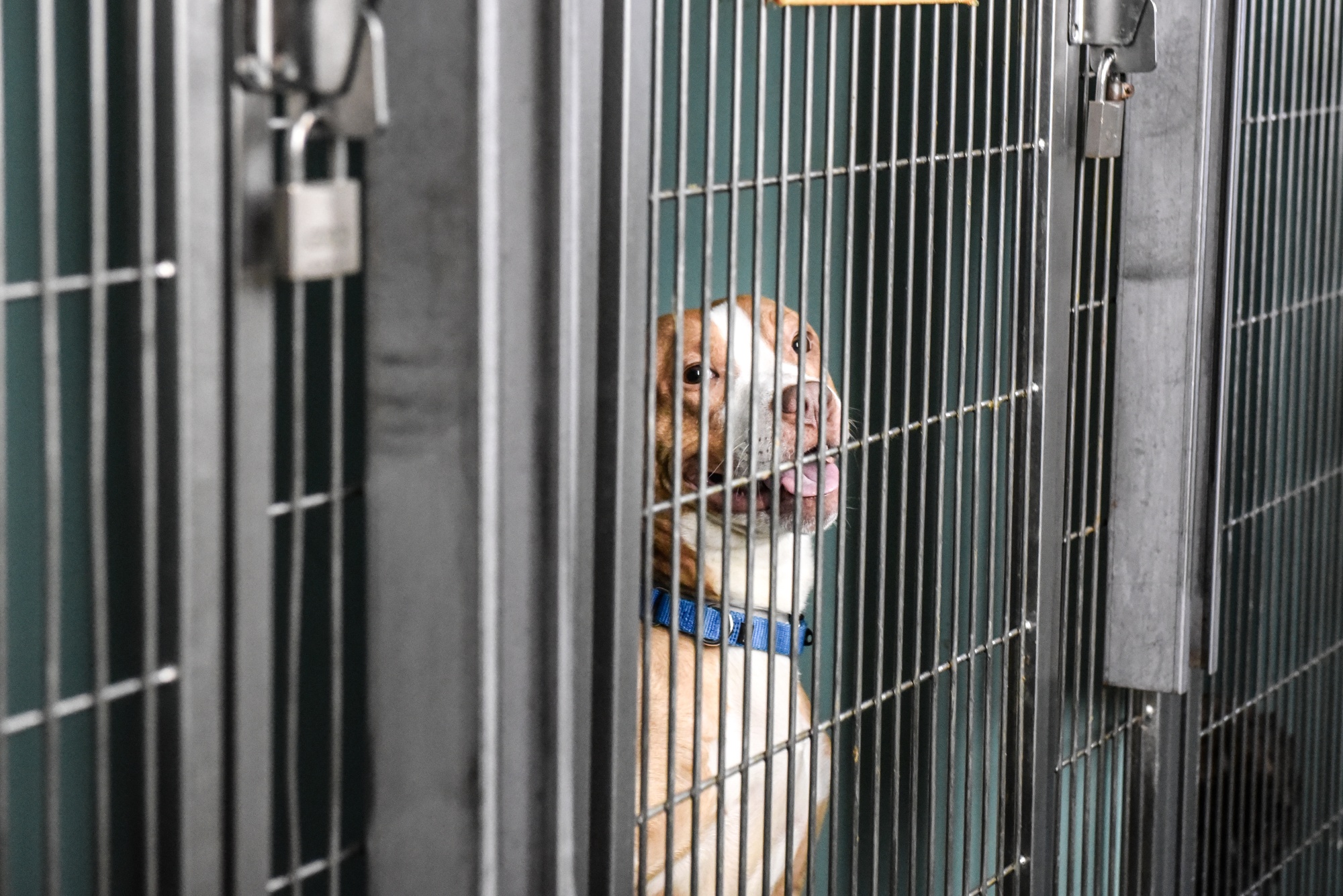This photograph, taken inside what appears to be an animal shelter, captures a heart-touching moment of a dog in a kennel. The setting is stark with gray metal cages, each secured with padlocks, and the central focus is on a light brown and white dog situated in the middle cage. The dog, wearing a blue collar, is looking directly at the camera with its mouth open in a smile-like expression, revealing a pink tongue. Its bright and alert eyes, coupled with its hopeful demeanor, create an impression that it is silently pleading for adoption. The dog’s attentive gaze and the inviting look on its face highlight its eagerness for companionship. Overall, this poignant image sheds light on the longing and vulnerability of animals in shelters, waiting for a loving home.